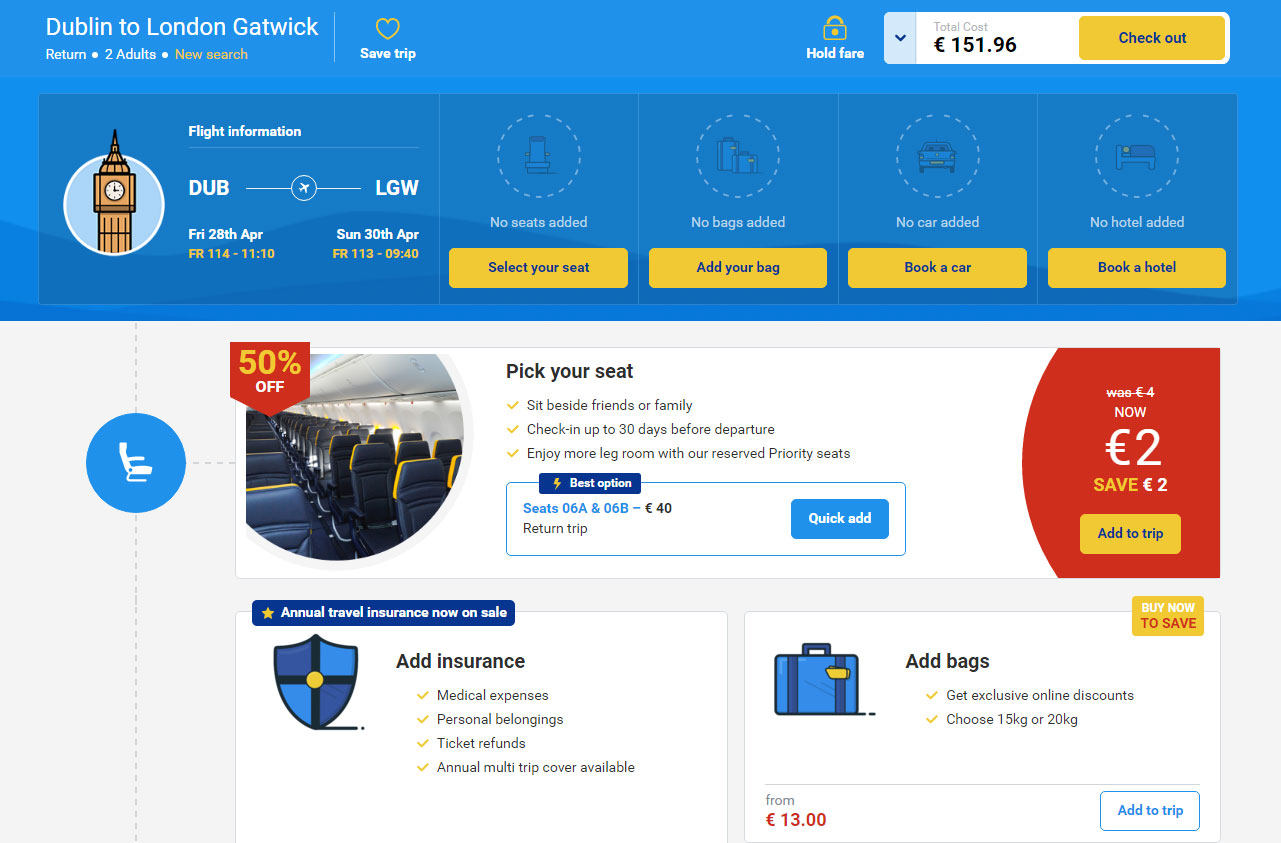This image, captured from a travel website, features a comprehensive flight booking screen. At the top, a periwinkle rectangle spans the width of the screen, with white text detailing the flight route: "Dublin to London Gatwick." Below this header, additional options are presented including "Return," "2 Adults," and "New Search."

The flight information is prominently displayed beneath the header, featuring the airport codes "DUB" connecting to "LGW" (London Gatwick) with an airplane icon between them. The departure date is clearly indicated as "Friday, 26th April," while the return flight is scheduled for "Sunday, 30th April." Underneath these details, the specific flight times are highlighted in yellow.

On the right side of the screen, a series of interactive yellow rectangular buttons invite users to customize their journey. These options include "Select Your Seat," currently marked as "No Seat Added," "Add Your Bag," and "Book a Car." Another option allows for hotel booking, providing comprehensive travel planning in one place.

Towards the bottom of the screen, a promotional banner advertises "50% Off," showcasing various airplane seats with a prompt to "Pick Your Seat." The promotion also mentions a savings offer: "Now 2 pounds, Save 2 pounds, Add Two Trips," encouraging travelers to make additional bookings.